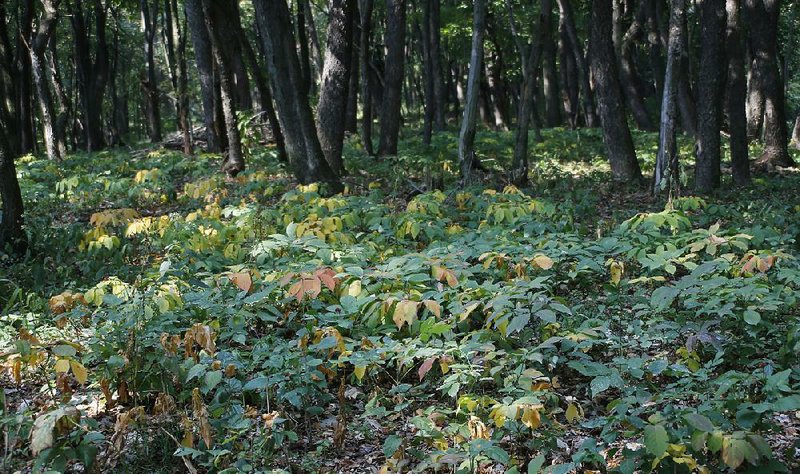The image portrays a vibrant forest scene with an array of vegetation. In the foreground, the ground is densely covered with lush green plants and short bushes, interspersed with leaves displaying a spectrum of colors—green, yellow, orange, and light brown. The background reveals a thick array of trees with dark brownish-gray trunks, creating a dense canopy. Sunlight filters through the trees, casting dappled light onto the foliage below, highlighting the vibrant, rich hues of the leaves. The overall setting is a sunlit forest, accentuating the natural beauty and diversity of the vegetation.